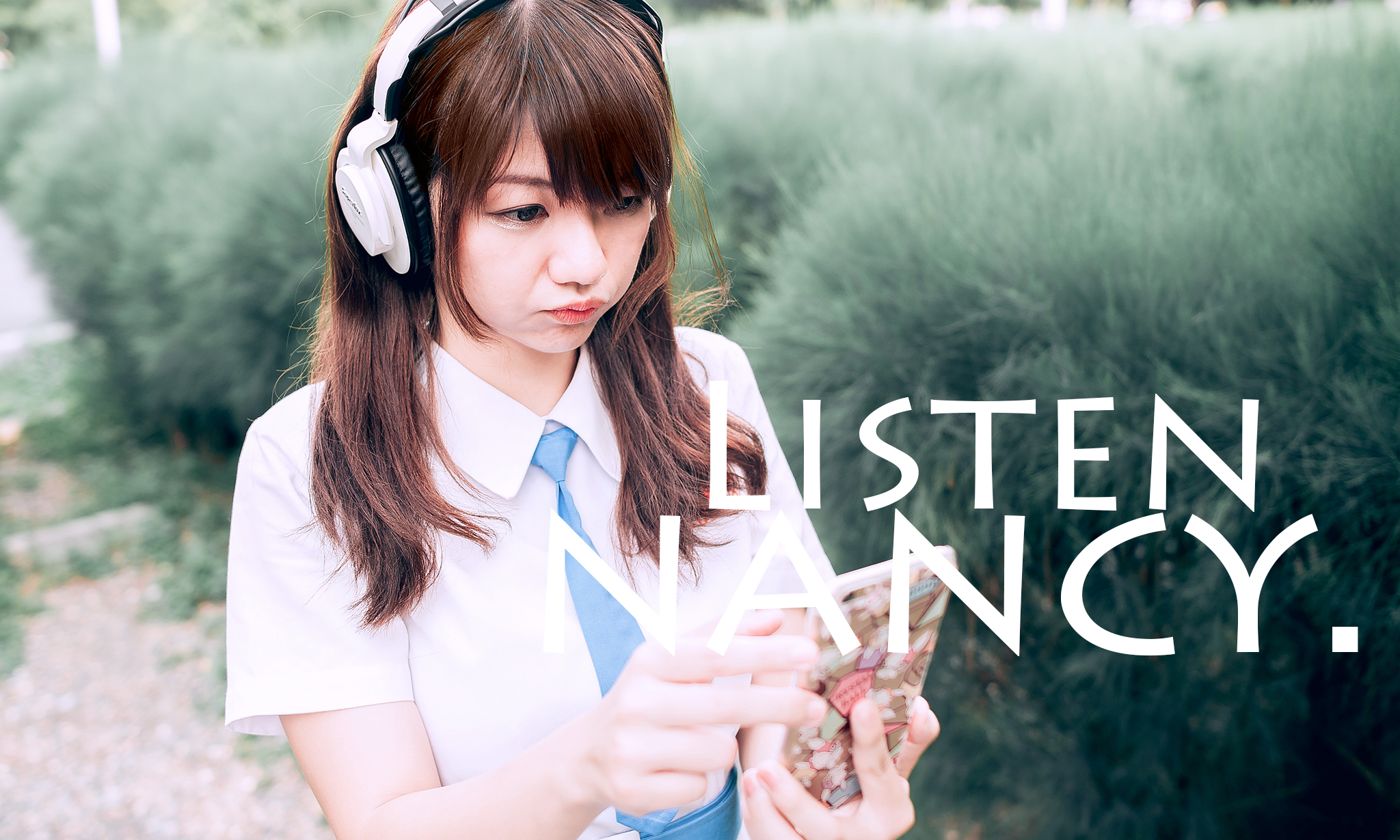This horizontal rectangular advertisement features a meticulously edited photograph of a young Asian girl, approximately 14 or 15 years old, with long dark hair highlighted brown. Her dark eyes are focused downward at her camouflage-patterned phone, suggesting she is engrossed in whatever she is listening to through her white earphones. She is dressed in a buttoned-up, short-sleeved white shirt paired with a light blue tie.

The blurred background comprises tall grasses and shoulder-high bushes of green and white hues, with white poles faintly visible in the farther left corner, possibly indicating a walkway. The ground around the bushes shows patches of dirt and grass. Overlaying the image on the lower right side, in white capital letters, the text reads, "LISTEN" in a smaller font, followed by "NANCY" in even bigger letters. The word "NANCY" spans part of the white area of the girl's shirt, making the first two letters slightly harder to distinguish.